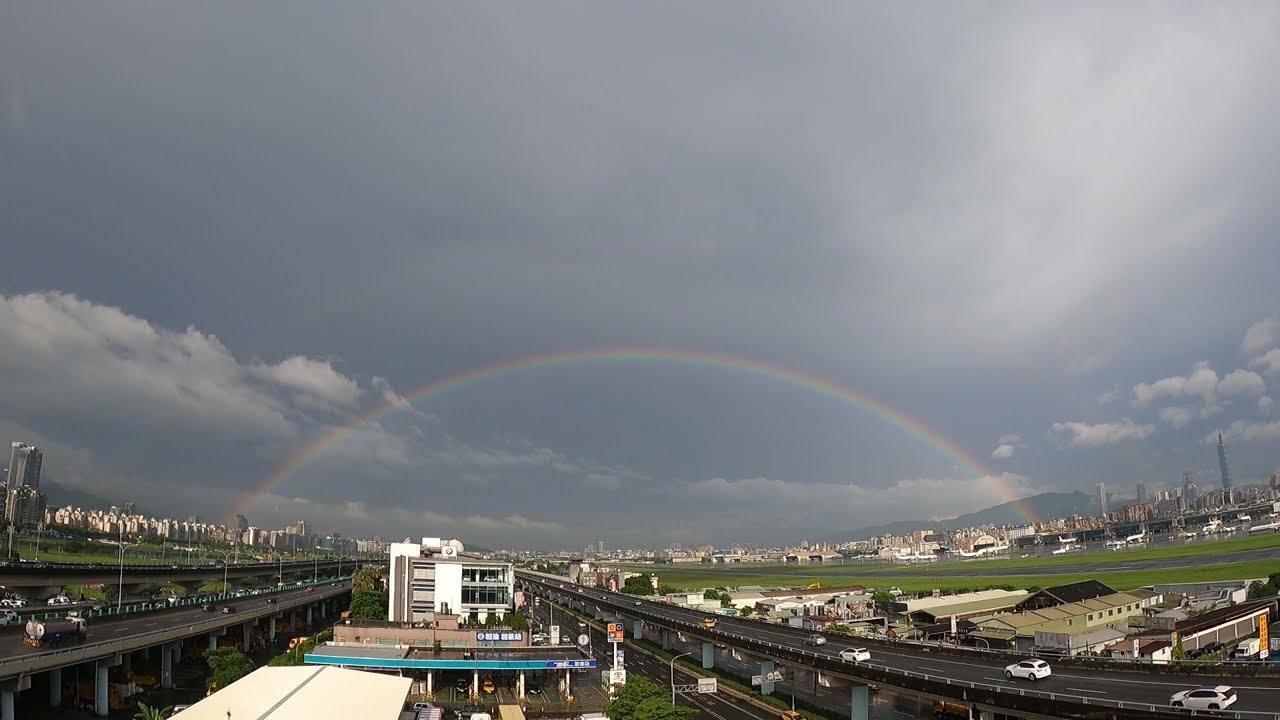The image captures an aerial view of a vast cityscape, showcasing a strikingly vivid, almost perfect rainbow arching majestically from left to right across the scene. The rainbow forms the centerpiece of the photograph, juxtaposed against a predominantly gray, cloud-filled sky. Below this natural spectacle, a sprawling urban environment unfolds, characterized by clusters of buildings scattered across both the far left and right sides of the image, emphasizing the city's extensive breadth. Prominent roadways and freeways, replete with cars, weave through the city, further highlighting the bustling urban life. Notably, a significant building in the middle of the frame displays Asian characters in blue and white, suggesting the city is in an Asian country. Grass patches and the distant silhouettes of mountains further enrich the background of this detailed urban tableau, with the interplay of dark clouds and the brilliant rainbow adding a dramatic visual contrast.